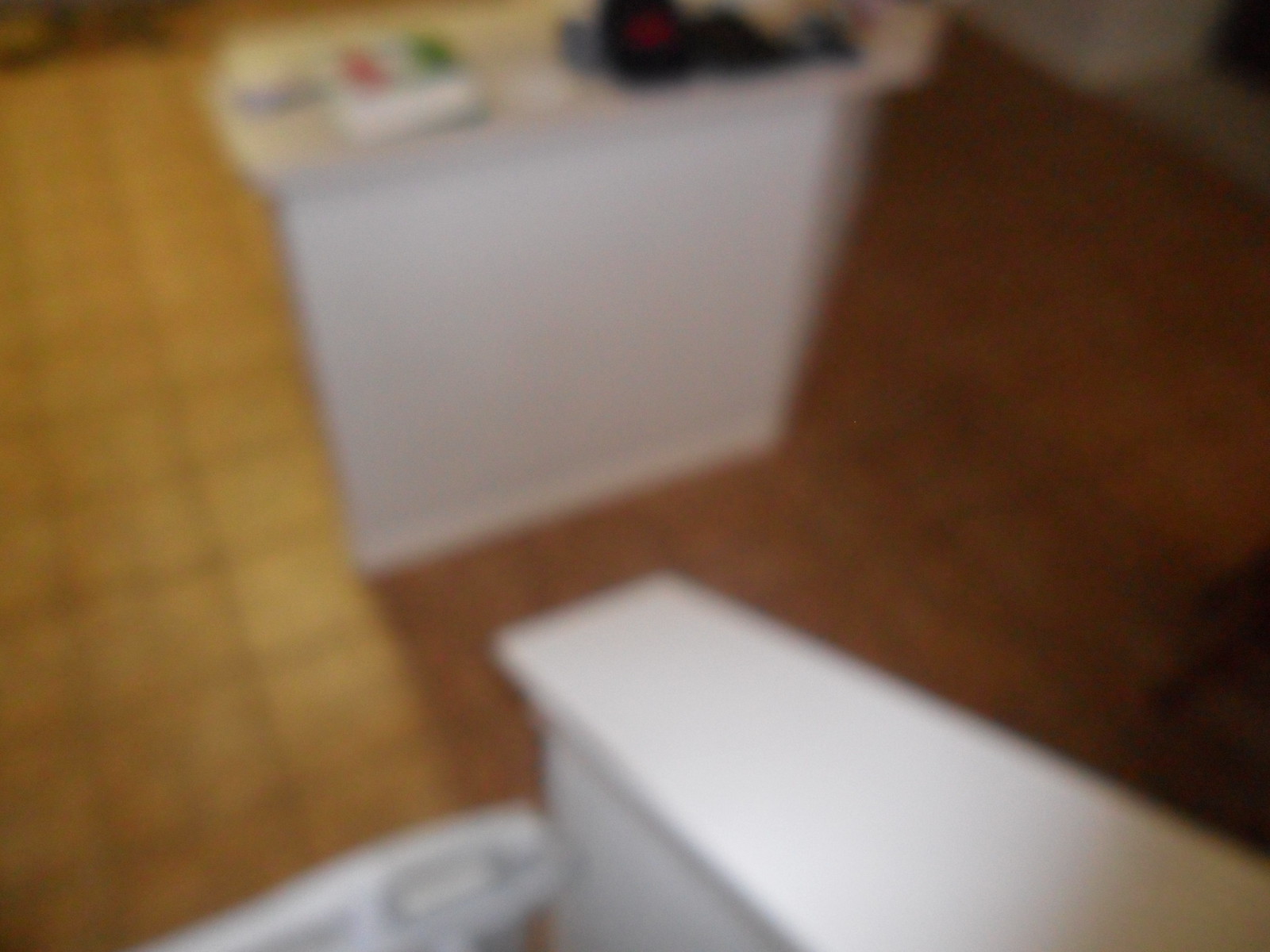This photograph, though blurry, captures an indoor kitchen scene from a top-down perspective. At the top of the image, a white countertop is visible. On the countertop are several objects, including a notable white item featuring a flag with red (or possibly orange), white, and green colors. To the right of this flag, there are darker, indistinguishable objects. The kitchen floor consists of square brown tiles, with a lighter hue on the left side of the photograph, seemingly illuminated by an orange light. In the bottom right corner, a white area is present, narrowing as it extends down, suggesting it might be an edge of a surface, appearing somewhat distorted. Positioned against this white surface to the left is another indistinct white object featuring bars, though the blur makes its exact nature unclear.